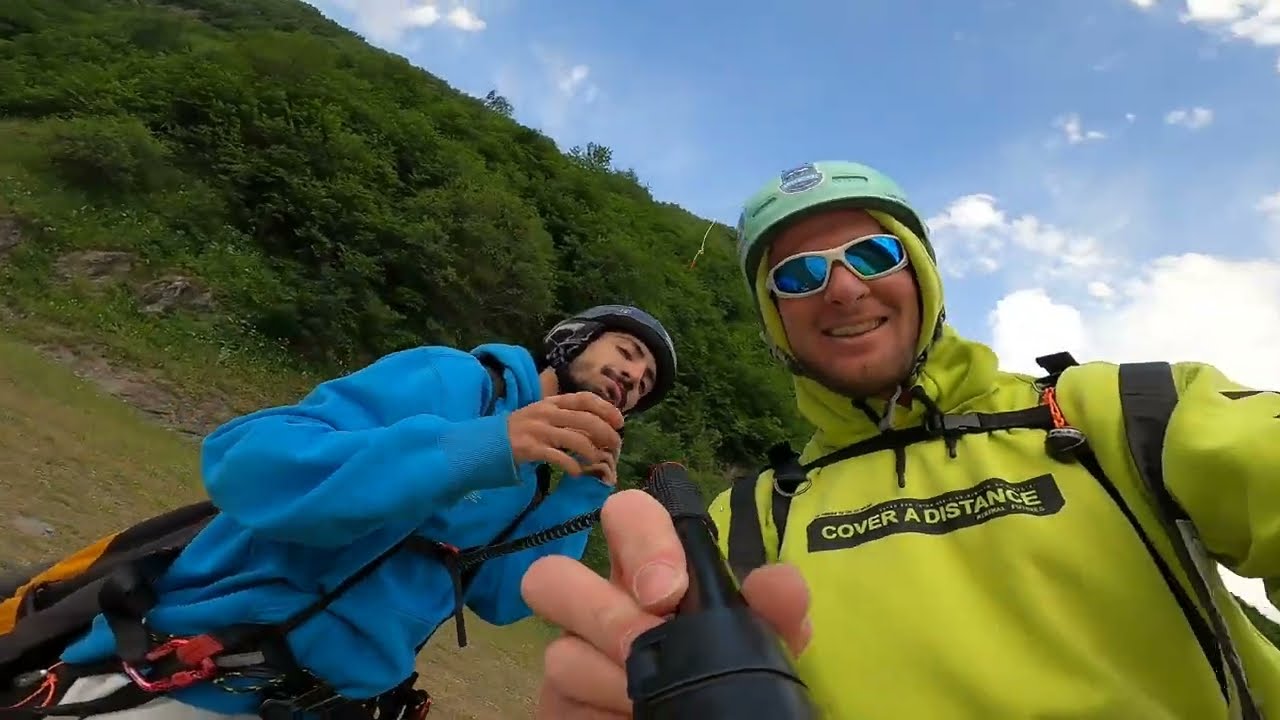In this detailed selfie, two men are depicted against a backdrop of a steep, green-vegetated hillside under a light blue sky with scattered white clouds. The man on the right, who might be holding the camera, sports a bright neon yellow hoodie with the words "Cover a Distance" on the front, the hood pulled up over his head. Over his hood, he's wearing a blue helmet with a white sticker on the front and is equipped with white-rimmed sunglasses featuring blue reflective lenses. His companion, on the left, has a mustache and beard and is dressed in a dark blue hoodie paired with white pants. He wears a dark blue helmet with a black strap and has carabiners attached to a belt, possibly indicating involvement in an activity like mountain climbing or bungee jumping. The perspective suggests the photo might have been taken with an action camera, possibly on a selfie stick, capturing the scene from a lower angle looking up at their smiling faces. The setting, complete with green shrubs and trees, the clear sky, and the vibrant colors of their gear, suggests a pleasant day spent engaging with nature, likely through adventurous outdoor activities.